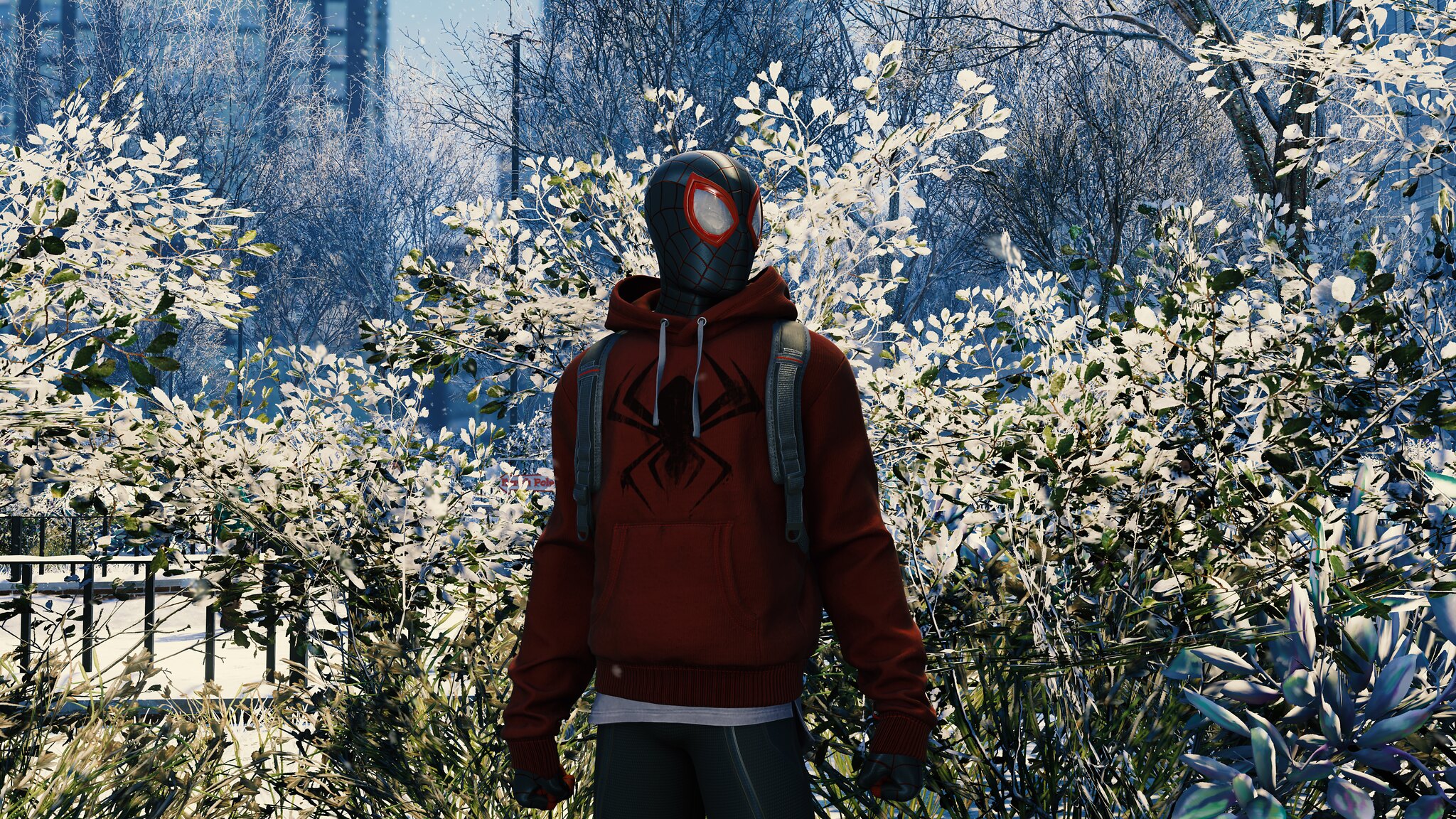In the image, Spider-Man is depicted wearing a distinctive black-brownish sweatshirt featuring an upside-down spider emblem on the front. The sweatshirt comes with a front pocket situated below the spider design. Straps from a backpack are visibly slung over his shoulders and extend underneath his arms, suggesting he is carrying essentials. Spider-Man's mask is colored in shades of gray to dark gray, with striking red accents around the eye areas. Complementing his look, he dons gray jogging pants. The setting appears to be an outdoor park filled with lush bushes and greenery. A building is partially visible on the left-hand side of the background, adding an urban touch to the natural surroundings. The overall scene captures a unique and detailed portrayal of Spider-Man blending into a park environment.